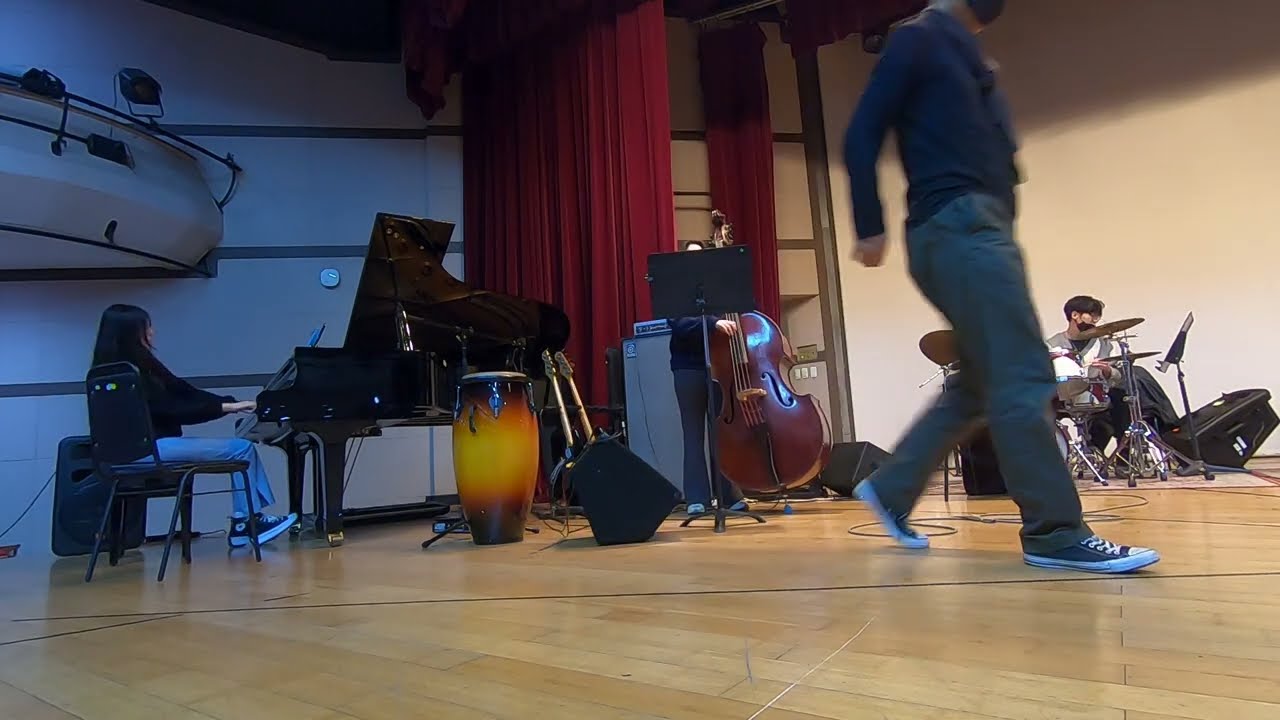In this detailed image of an indoor music room, akin to a recording studio or gymnasium set up for band practice, a hardwood floor typical of a basketball court stretches across the scene. The environment is bathed in diverse colors, including light brown, black, blue, orange, tan, red, maroon, gray, and silver. A large white wall, trimmed in a blue or brown tone, occupies the background, with a notable semi-circular balcony hosting mounted stage lights above.

Various students are scattered around, engaging with different musical instruments. To the left, a woman with long dark hair, dressed in jeans and a dark shirt, is seated at a large black upright piano, with a black speaker positioned behind her. In front of her on the floor lies a drum and a couple of music stands supporting guitars. Near the center-right, a man in cargo pants, a blue shirt, and Converse sneakers walks by, drawing attention with his casual stride.

Adjacent to him, a man absorbed in drumming sits at a drum set complete with cymbals and a black mask over his face while reading from a music stand. Off to the right, another individual stands behind a double bass, supported by its own music stand. Instruments are central to this lively scene, with bongo drums, a bass, and several guitars lying on the floor, showcasing a thorough setup for a dynamic band practice.